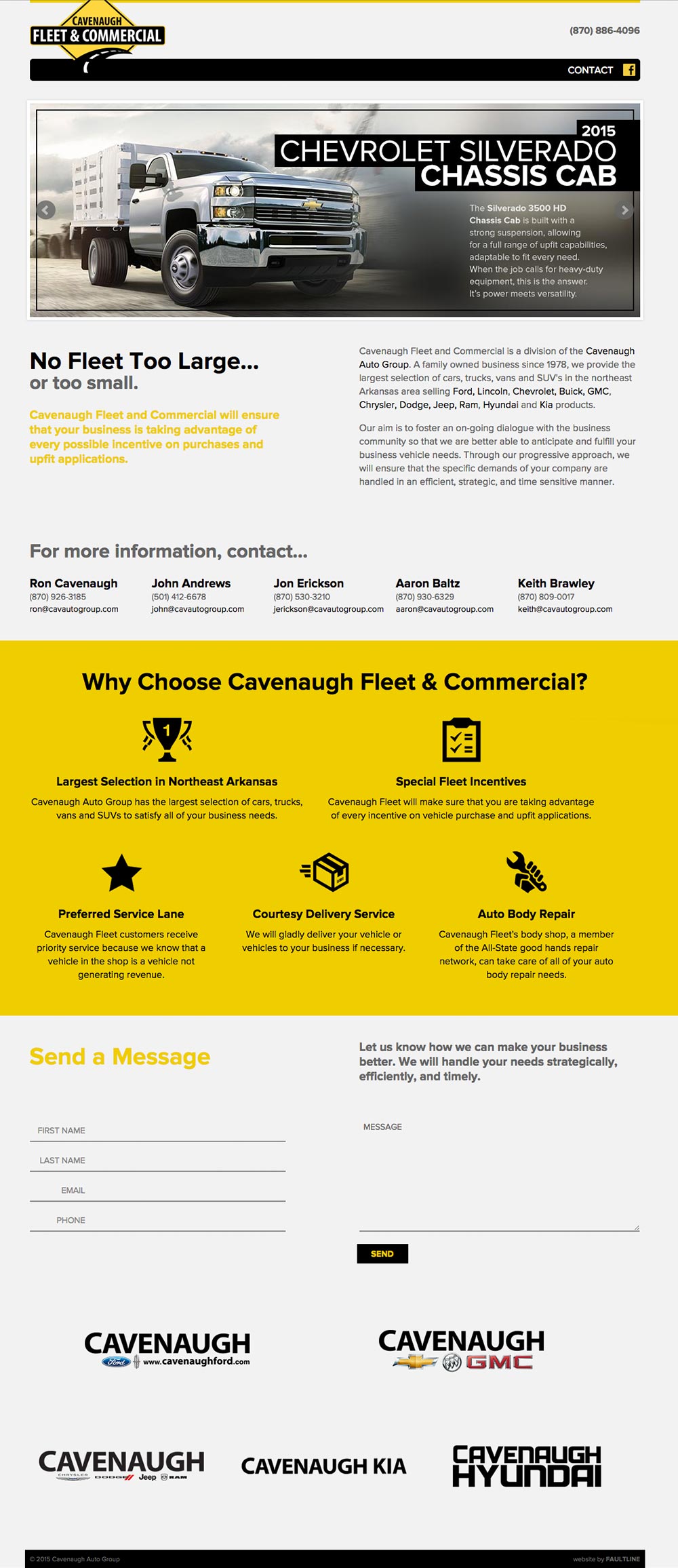The advertisement features a well-structured layout for a Chevrolet Silverado Chassis Cab. At the top, a black rectangular box with "Fleet and Connection" written inside is superimposed over a gold diamond-shaped background. Directly beneath this, a black bar containing a search function is prominently displayed. The main image shows the Chevrolet Silverado truck set against a sophisticated gray-white backdrop.

The advertisement includes a description reading, "No fleet too large or too small," presented on a light gray background, followed by a brief narrative. For further details, viewers are instructed to contact the relevant representatives, with specifics listed for five categories of contacts, each accompanied by a phone number.

A gold box highlights reasons to choose Cavanaugh Fleet and Commercial, embellished with icons such as an award, a star, a box, and a tool, each with corresponding descriptions beneath. Another light gray section invites users to send a message by providing their information. The ad also includes mentions of related dealerships: Cavanaugh GMC, Cavanaugh Hyundai, Cavanaugh Kia, and possibly another Cavanaugh outlet, though the text is too small to read.

This detailed and organized layout emphasizes essential information about the Chevrolet Silverado Chassis Cab and provides clear instructions for potential customers to reach out and learn more.